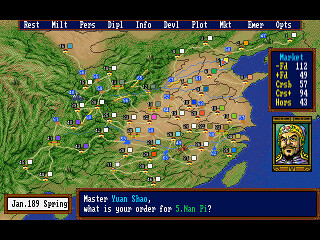The image appears to be a screenshot from a strategy video game. The player's perspective is a bird's eye view of a lush coastal landscape, possibly an island or a shoreline. In the lower part of the screen, the text "January 189 Spring" is displayed, setting a historical or seasonal context. A dialogue box in the middle of the screen reads, "Master Yuan Shao, what is your order for five-man pie?", indicating a command or dialogue within the gameplay. The landscape showcases greenery and various colored squares that likely represent different characters or units. Across the top of the screen, a menu with various options—labeled as "Best Mints," "Pearls," "Info," "Devil," "Plot," "Emergency," and "Options"—suggests interactive elements and actions the player can take. The rich details and interface elements highlight the strategic and immersive nature of this game.